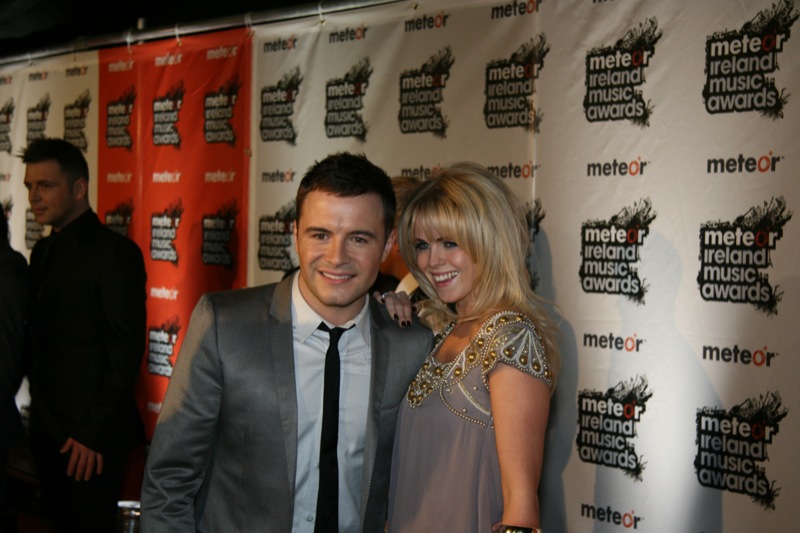The image captures a nighttime scene outside at the Meteor Ireland Music Awards. A young man and woman are posing and smiling for the camera in front of a press banner adorned with multiple logos for the event. The man is dressed in a dark gray suit jacket paired with a thin black tie and a white button-up shirt. He has short dark hair, styled primarily on top of his head, and he is smiling. Next to him stands a woman with long blonde hair cascading down her back. She sports a gray dress featuring short sleeves adorned with intricate gold embellishments and white accents on the shoulders and chest. In the background, you can see another man in a black suit jacket facing a different direction, seemingly taking photos, along with other individuals further along the press banner, all adding to the bustling atmosphere of the awards ceremony.